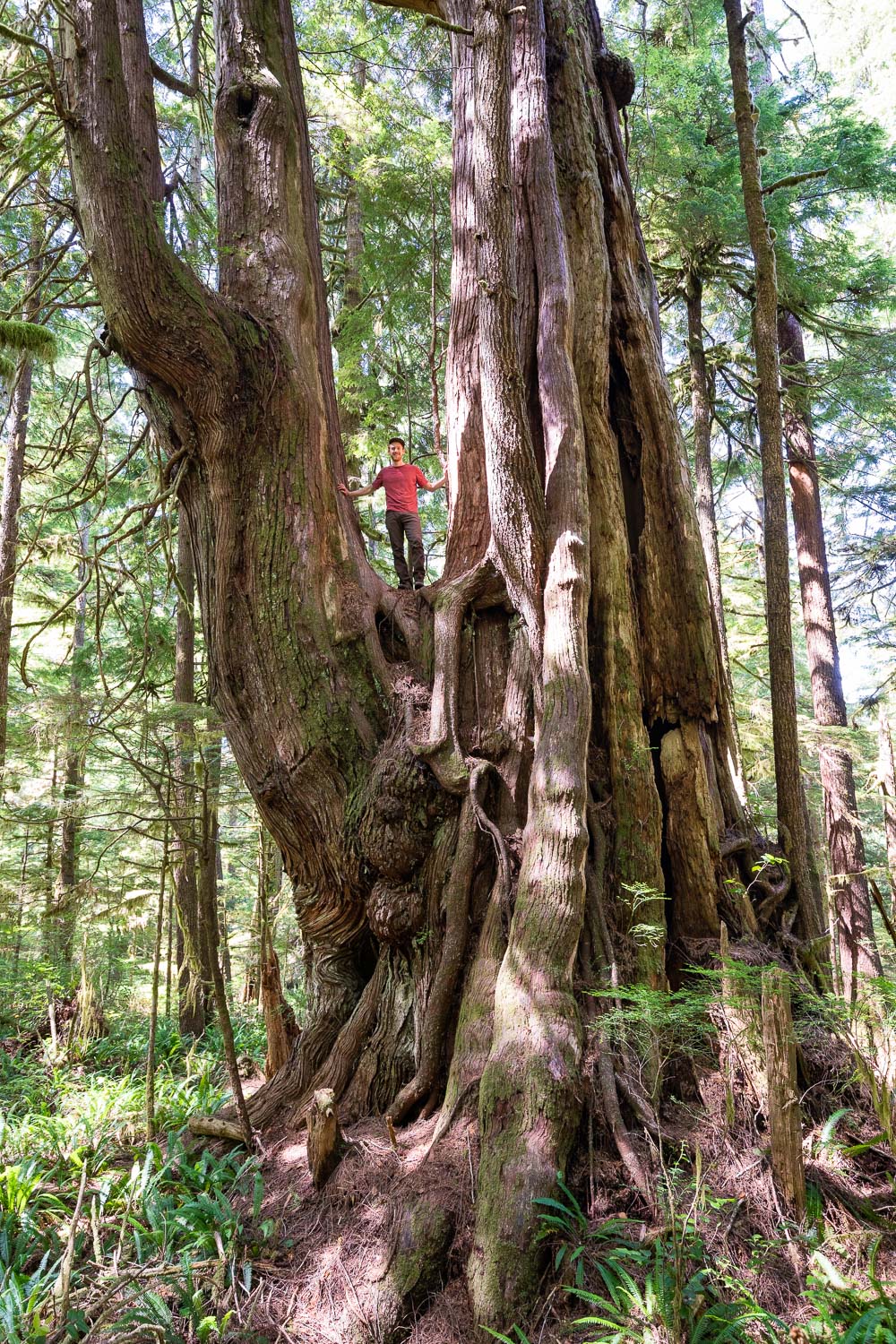This is a daytime photograph set in a dense forest, with the main focus on a colossal tree, approximately 20 to 30 feet tall, that prominently splits into a U-shape. Surrounding this giant are numerous smaller, tall trees, their tops extending beyond the frame, and high leaves indicative of a lush forest environment. Standing in the crook of the split trunks is a young man with short dark hair, wearing a short-sleeved red shirt and brown pants. The man, who appears to be white, has placed his hands on the side branches of the tree and is looking directly at the camera. Dappled sunlight filters through the canopy, illuminating parts of the tree bark and revealing the verdant, leafy forest floor below.